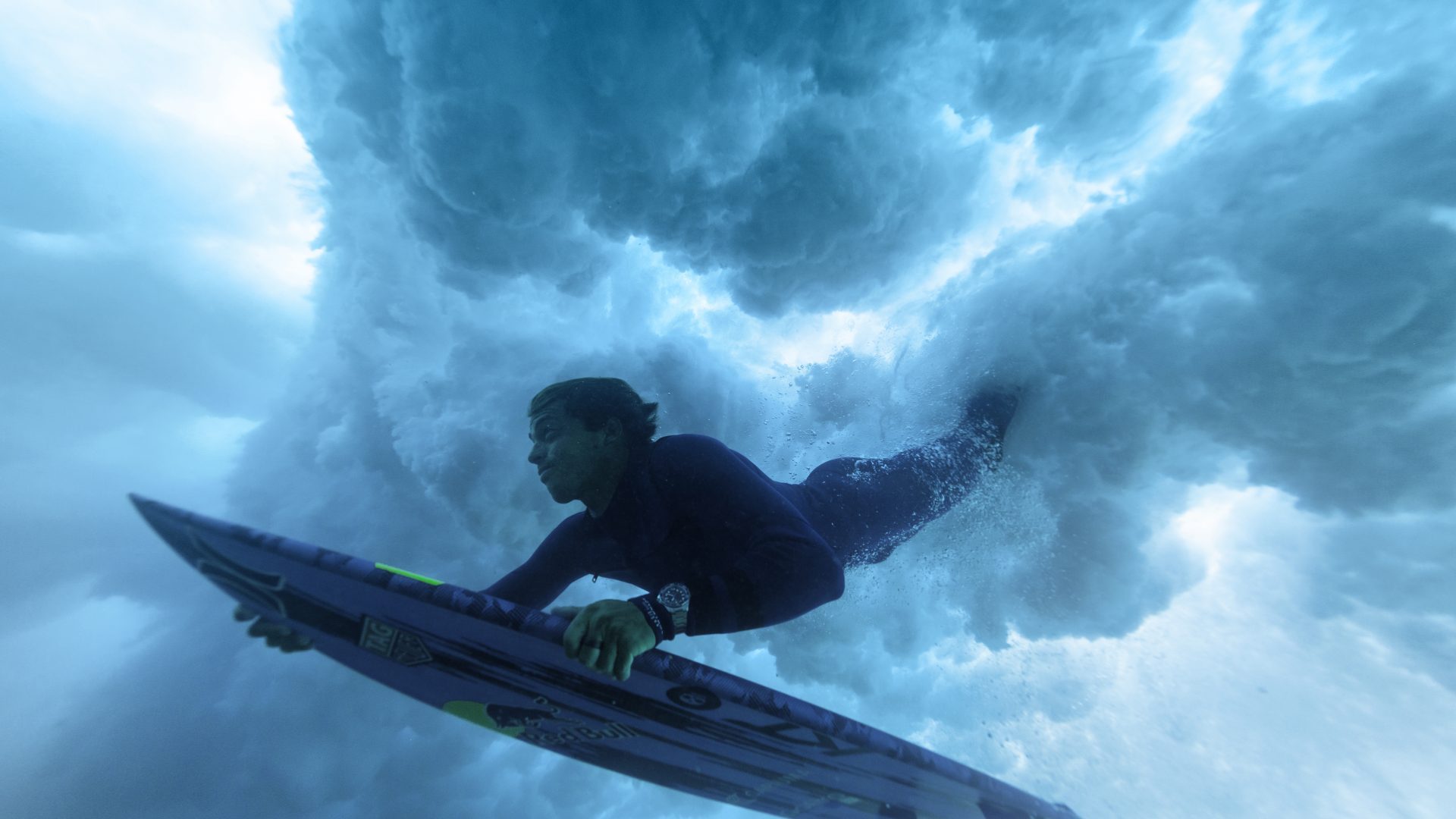The underwater photograph captures a moment of serene intensity as a surfer, dressed in a black wetsuit and wearing a mechanical watch, is surrounded by the churning, cloudy blue waters of a wave. The surfer is horizontally aligned with his body extended, firmly grasping his surfboard which is positioned below him. His calm demeanor contrasts with the turbulent, foam-filled water above that resembles billowing, fluffy clouds. The image's composition emphasizes the contrast between the darker blue wave embracing the surfer and the lighter, frothy sections that frame the scene, creating a striking and dynamic underwater spectacle.